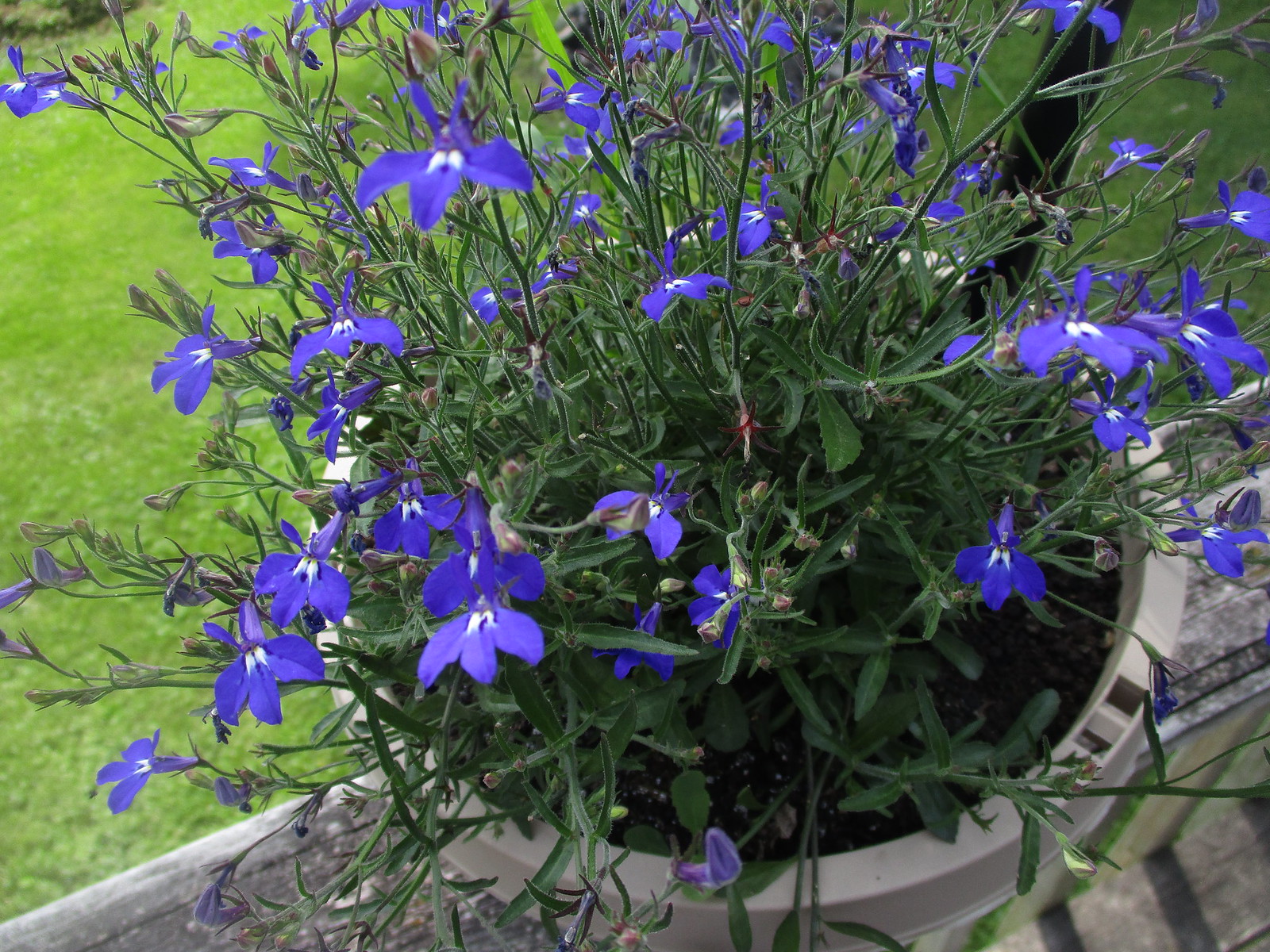This detailed image captures a vibrant outdoor garden scene, centered around a gray heavy-duty plastic planter pot filled with lush green stems and numerous small, thin-petaled, bright purple flowers, each with a distinctive white center. The photograph is taken from an overhead perspective, highlighting the arrangement of the flowers and the dark brown soil mixed with white speckles. The pot rests on a weathered wooden surface, likely part of a porch railing, with additional slats and a similarly aged wooden floor visible beneath. The background features a broad, brightly lit, closely mowed green lawn, with a slight gradient suggesting shading or variations in grass color. The scene appears to be an outdoor garden or balcony area, captured in broad daylight without any text or signage present.